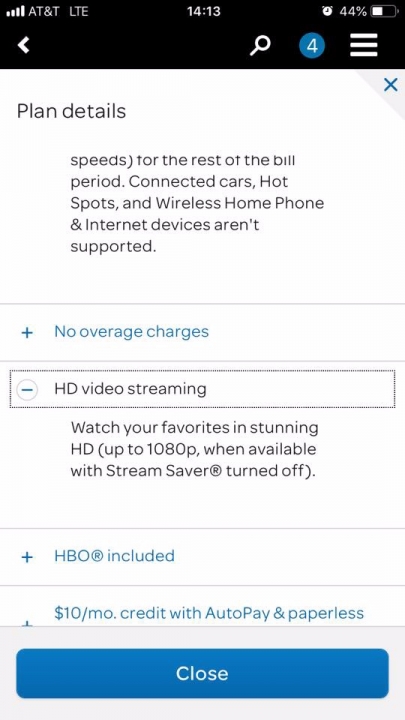This screenshot depicts detailed information from an AT&T mobile device, including service status, device details, and plan information. The device currently has full signal strength, indicated by four bars, and is using LTE data. The network provider is AT&T. It is 14:13 on the device's clock, and the battery is at 44% charge with an alarm set, as denoted by the alarm icon.

At the top of the screen, navigation options include a back button on the left, a magnifying glass icon for search, and a numerical indicator showing four notifications. There's also a menu bar represented by three horizontal lines, and an X button in the top right corner, likely to exit this page.

The page header reads "Plan Details," outlining the specifics of the current billing period. It's noted that speeds for this period are as follows: connected cars, hotspots, wireless home phones, and internet devices are not supported. There's an expandable section indicated by a plus sign titled "No coverage changes," meaning no changes have been made to the service coverage.

Beneath that header, there is another section, currently expanded, for HD video streaming, which is marked by a negative sign that would collapse the section. This section explains that users can stream their favorite content in stunning HD up to 1080p when Stream Saver is turned off.

Additional plan perks are listed in blue text:
- HBO included
- $10 a month credit with AutoPay and paperless billing
- No overcharges
- HBO included again (likely a repetition error)
- $10 a month credit (another repetition)

Most of the text within this screenshot is black, outlining the general information about the plan, while specific benefits are highlighted in blue text to draw attention.